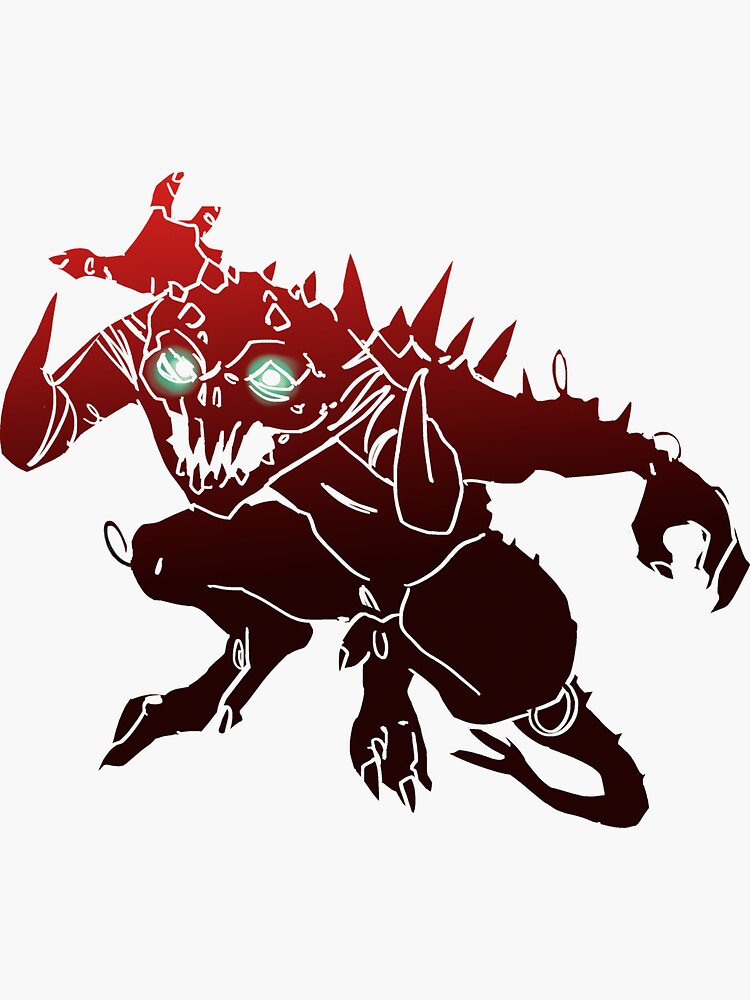This highly detailed image portrays a menacing, fantastical monster on a light gray background. The creature's upper half is maroon red, transitioning to a dark black or brown lower half. Its glowing, triangular eyes are blue with white circular centers, casting an eerie light. The monster's mouth is open wide, displaying an array of large, sharp teeth, including four prominent upper fangs against a white background.

The monster has an angular, spiky appearance, with red spikes lined in white adorning its head, shoulders, and back, among which five are distinctly prominent. Its arms and legs are armed with razor-sharp claws, with one arm ending in a hook-like claw. White lines traverse the creature's body, accentuating its limbs and tail, which is shaped like a lizard's with a forked end.

Weird extensions and white loops are visible around its limbs, adding to its bizarre anatomy. Notably, the right knee and left forearm feature swirling extensions, completing the surreal and terrifying visage of this otherworldly being.